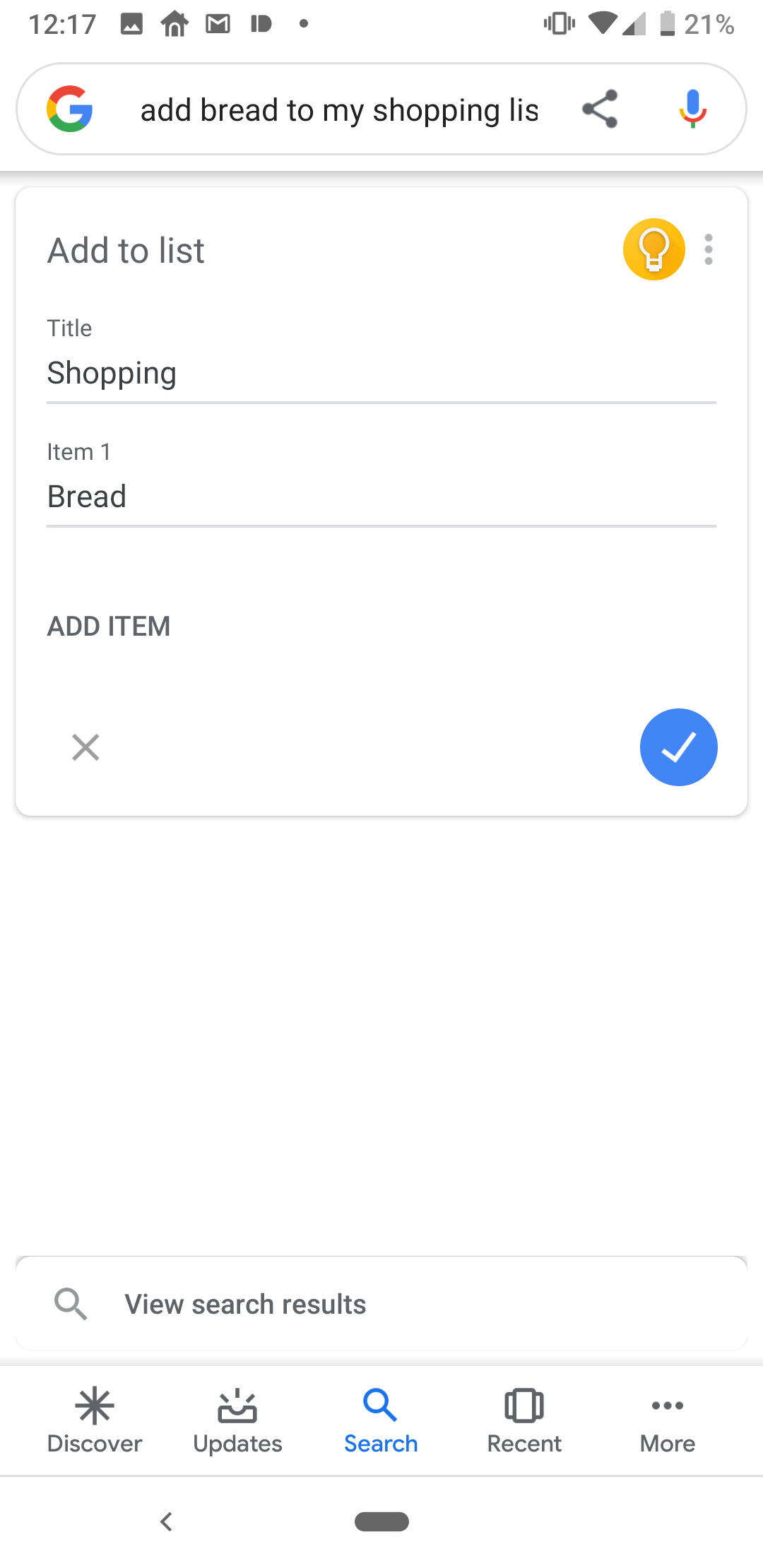Here's a detailed, cleaned-up caption for the image:

---

This screenshot, likely taken from a Samsung or non-Apple device, shows various elements of its user interface. At the top of the screen, the time reads 12:17, flanked by several icons: a picture icon, a house icon, a Gmail icon, an unidentified icon resembling a bullet pointing right, a dot, a toggle icon, a fully filled Wi-Fi icon, a signal bar at nearly half strength, and a battery icon indicating 21% charge.

Below the top bar, an oval-shaped Google search bar features the colorful "G" logo in red, yellow, green, and blue, along with the text "Add bread to my shopping list." This bar also includes a share icon and a colored microphone icon. 

Further down, there's a squared section. The upper left of this section displays "Add to list," while the upper right shows a yellow circle with a light bulb in it, alongside three vertical dots. The left side underneath this area reads "Title" followed by "Shopping." A thin gray line separates this from the list section, where "Item 1: Bread" is listed under another thin gray line. Below that, there's an "Add item" prompt with an "X" on the lower left and a blue circle featuring a checkmark on the right.

At the bottom of the screen, a navigation bar includes buttons for "Discover," "Update," "Search," "Recent," and "More," each with its corresponding icon.